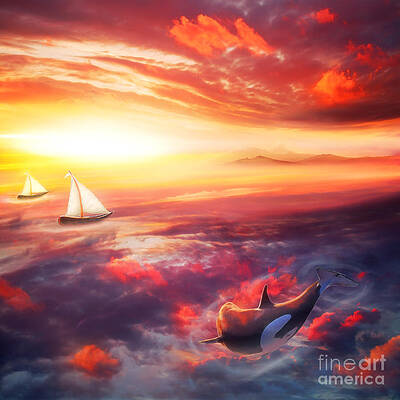This vibrant artwork captures a dramatic sunset at sea, characterized by a spectrum of colors ranging from deep red and orange to purple and dark blue. The scene is dominated by a dynamic depiction of an orca whale breaching the wild, choppy waters, creating splashes and ripples. The sky and ocean reflect an intense blend of fiery hues, enhancing the vibrant and almost surreal atmosphere. In the background, towards the left, two small sailboats with white sails float on the waves, one further in the distance than the other. A hint of mountainous landscape peeks through the clouds on the right. A watermark in semi-transparent white text, in Century Gothic font, reading "Fine Art America," is visible in the bottom right corner, indicating the artwork's origin.